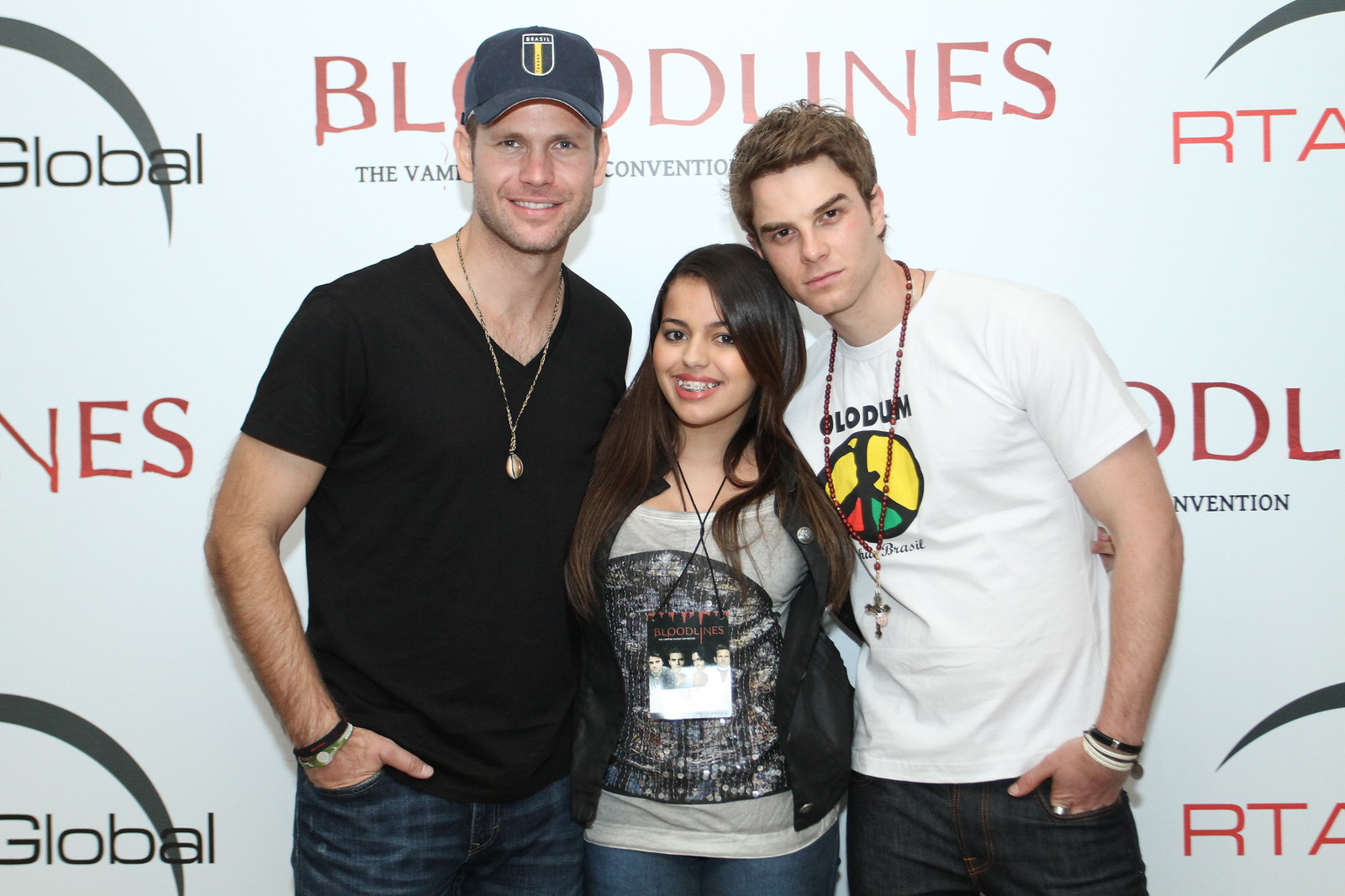In the photograph, three people stand in front of a tall white wall covered with multiple logos, prominently featuring a red font mimicking dripping blood that reads "Bloodlines" with "The Vampire Convention" in black text below, and another logo with "RTA Global" in red and black, intersected by a semicircle line. In the center of the image, the group is composed of a man on the left, a woman in the middle, and another man on the right.

The man on the left is dressed in blue jeans and a black, short-sleeve v-neck t-shirt. He accessorizes with a blue baseball cap that has a yellow and gray logo on the front, and a long gold necklace with a round pendant. He also wears two bracelets—one black, one green—and has a fair complexion with blue eyes, visible facial stubble, and a broad smile. His hand rests casually in his pocket.

In the center stands a woman with long dark brown hair, adorned with peach-colored lipstick and braces. She is wearing a gray t-shirt that appears to have sequins and a lanyard around her neck, which features the "Bloodlines" text. She also has on blue jeans and is smiling.

To the right is a man with brown hair, clad in dark-colored jeans and a white t-shirt. A long necklace with a cross hangs around his neck. He stands closely beside the woman in the middle, completing the trio against the logo-covered wall, suggesting they are attendees or participants at a vampire-themed event.